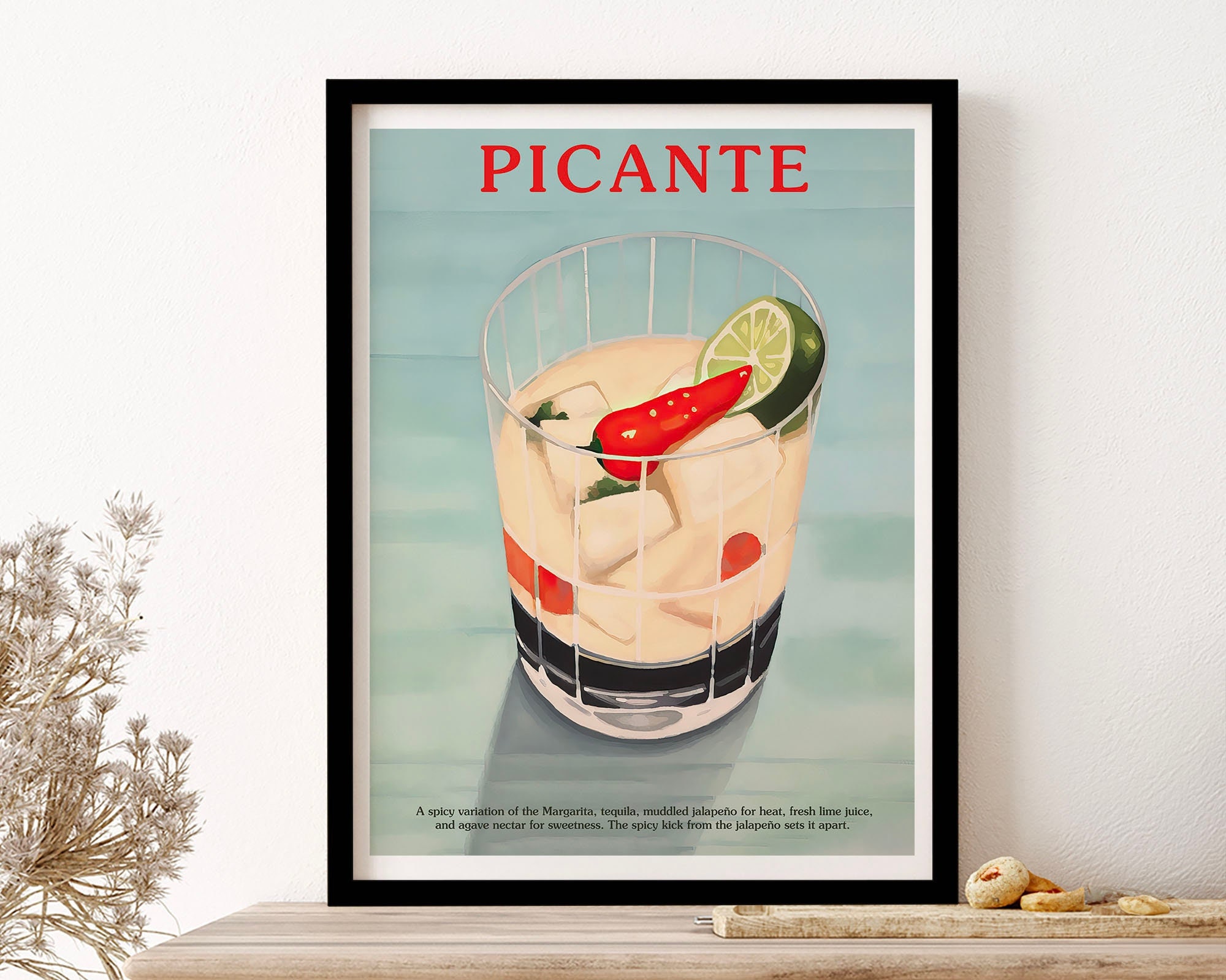This photograph showcases a framed poster titled "PICANTE" in bold red font at the top. The image within the black frame, with a white mat border, exhibits a light blue and hazy gray background with subtle lines. Central to the illustration is a clear glass containing a light tan liquid, indicative of a margarita on the rocks. The drink features visible ice cubes, a red pepper, and a lime wedge. The caption at the bottom describes the drink as "a spicy variation of the margarita" made with tequila, muddled jalapeno for heat, fresh lime juice, and agave nectar for sweetness, emphasizing that "the spicy kick from the jalapeno sets it apart." The framed poster is set against a white wall, resting on a natural wood table. Adjacent to the poster on the right side appears to be a brown plant, and there is mention of bread and plants on the table, adding to the indoor setting's cozy ambiance.